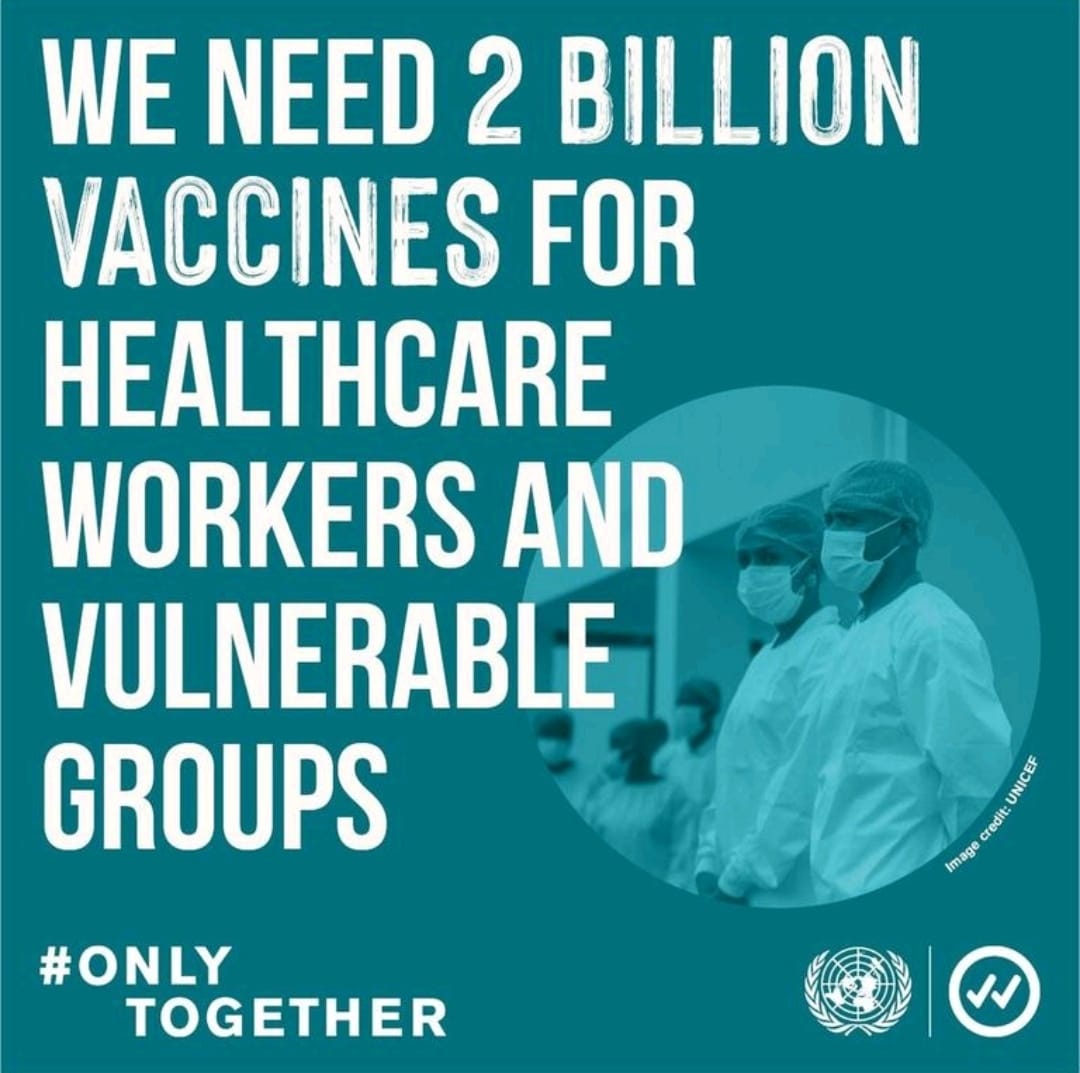The image features a teal square with prominent white text in all capital letters reading, "WE NEED 2 BILLION VACCINES FOR HEALTHCARE WORKERS AND VULNERABLE GROUPS." The numeral "2" is used instead of the word "TWO." In the lower right section of the square, overlapping slightly with the text, there is a smaller, brighter teal circle. Inside this circle, there is an illustration of five healthcare workers shown from the waist up, all wearing scrubs, headgear, and face masks.

Below the illustration, there is a label that reads, "Image Credit: UNICEF." In the bottom left corner of the image, the text "#ONLY TOGETHER" is displayed. The hashtag is on the first line next to the word "ONLY," and "TOGETHER" is written on the second line starting at the letter "O" in "ONLY."

On the right side of the image, there is another circle featuring an emblem consisting of a stylized wreath of wheat on both sides. Within this circle, there is a thicker white outline and two check marks placed side by side.